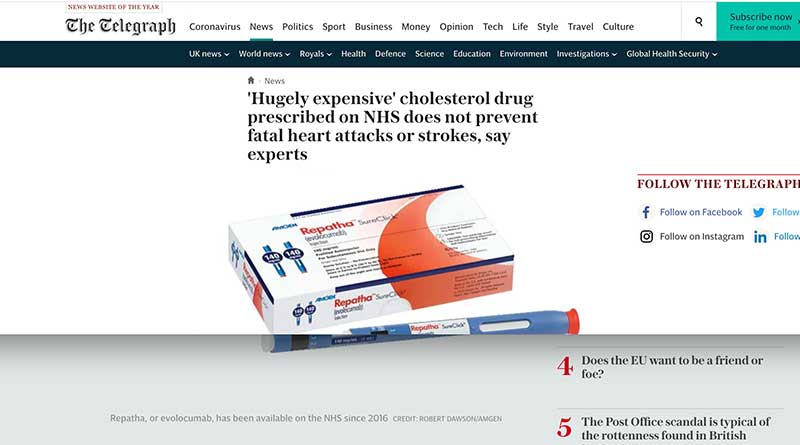This image appears to be a screenshot from a news website, set against a white backdrop. In the upper left-hand corner, there's red text that appears blurry but seems to say "News Something of the Year." Directly below in newspaper-style print is "The Telegraph." 

To the right of these, the site features several section titles in black: "Coronavirus," underlined with a green bar, and then "News," "Politics," "Sport," "Business," "Money," "Opinion," "Tech," "Life," "Style," "Travel," and "Culture" arranged horizontally. There is also a black hourglass icon signifying search functionality, and next to it, a small green box that says "Subscribe Now" in black, with a subtext "Free for one month."

Below, a blue bar spans the center of the page, featuring white text listing more categories from left to right: "UK News," "World News," "Royals," "Health," "Defense," "Science," "Education," "Environment," "Investigations," "Global Health Security," each accompanied by a white drop-down arrow.

Centered below these categories is a home icon and the word "News" in black. Underneath, a headline in black reads “‘Hugely expensive’ cholesterol drug prescribed on NHS does not prevent fatal heart attacks or strokes, say experts.” Beneath this is an image of a medicine box marked "REPATHA" in red in the upper left corner. The box contains what appears to be an injection pen with a blue body and red cap, resembling an insulin pen for self-injection.

On the right-hand side of the page, there's a section titled "Follow The Telegraph" with prompts to follow on Facebook and Instagram. Additionally, a red number "4" is noted in the bottom right-hand corner with the adjoining text: "Does the EU want to be a friend or foe?" followed by a red number "5" and the text: "The post-office scandal is typical of the rottenness found in British...". 

The detailed layout of text, icons, and images suggests a comprehensive and varied news website offering extensive information across numerous categories.